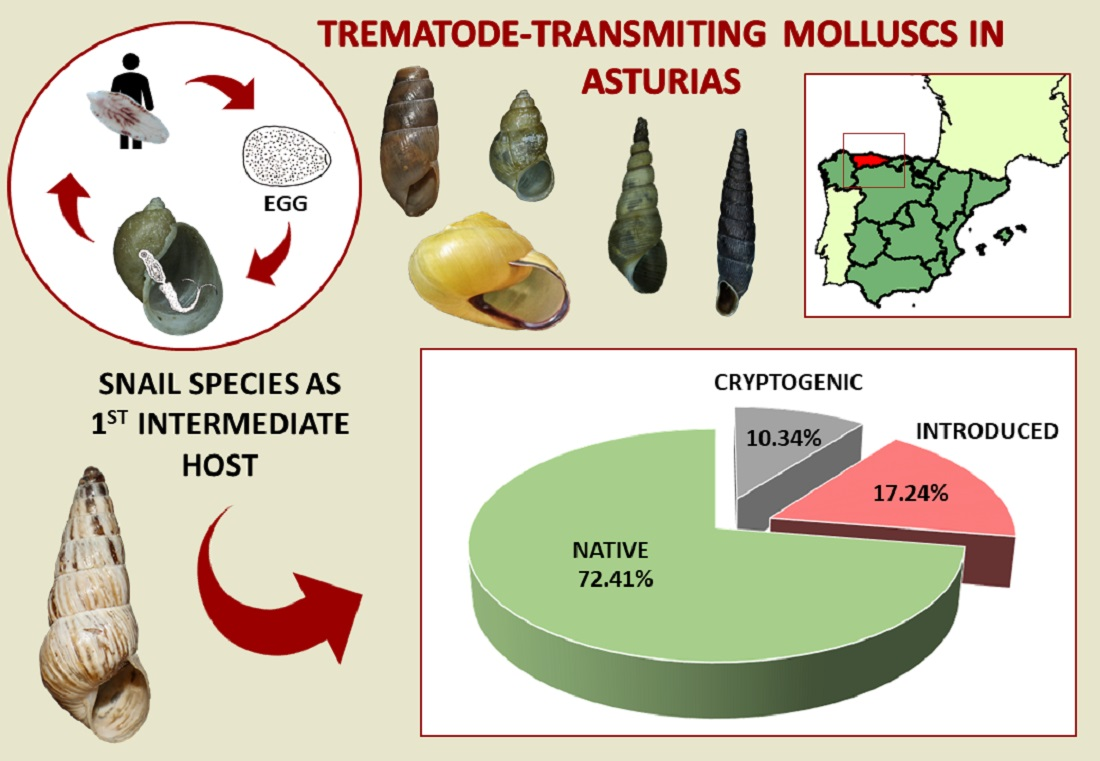The image is a detailed infographic titled "Trema Toad Transmitting Mollus in Asteris," written prominently in red at the top. Below the title, there are five snail shells displayed in a range of colors from dark brown to yellow. On the right-hand side, there is a circular diagram showing a transmission cycle, starting with a person, followed by arrows leading to an egg, and then into a shell containing a tadpole-like form, before returning to the person. Adjacent to this diagram, a small green map with a red square highlights a specific region. Below the map, a pie chart shows snail species distribution: a large green section labeled 'Native 72.41%', a red section 'Introduced 17.24%', and a gray section 'Cryptogenic 10.34%'. To the left of the pie chart, text reads "Snail Species as First Intermediate Host." The infographic background is beige, with prominent colors including green, red, and the varied hues of the snail shells.